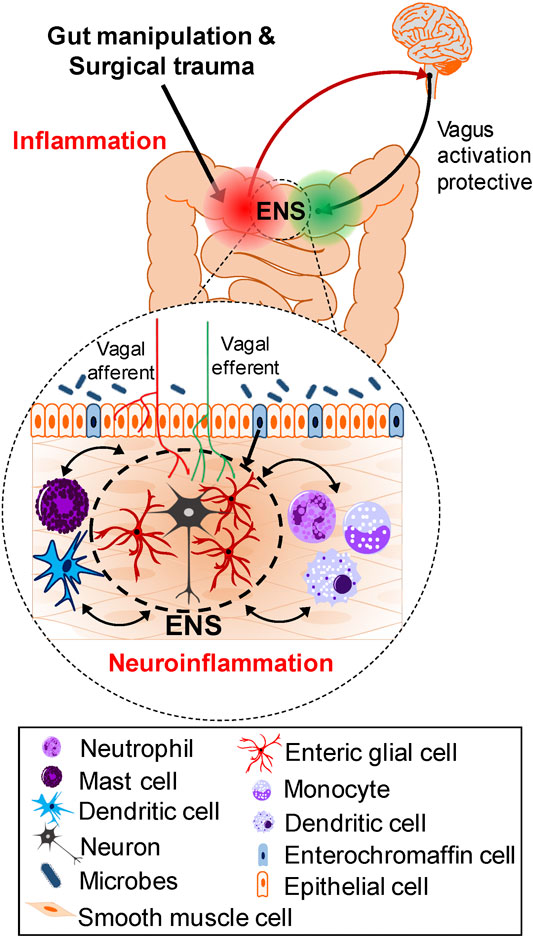This detailed medical diagram, resembling an illustration from a textbook, is centered on gut manipulation and surgical trauma. The image prominently features the intestines alongside a brain, connected by arrows illustrating various physiological responses. Key areas are highlighted in red and green, indicating inflammation and vagus activation, respectively. Additional labels include ENS, vagal afferent, vagal efferent, and neuroinflammation, signifying complex interactions between the gut and nervous system. A blow-up section within a circle further examines these processes, providing insights into cellular interactions. This section, demarcated into vagal afferent on the left and vagal efferent on the right, shows various cell types within the intestines. A comprehensive key at the bottom deciphers the symbols, identifying neutrophils, mast cells, dendritic cells, neurons, microbes, smooth muscle cells, enteroglial cells, monocytes, enterochromaffin cells, and epithelial cells, offering a thorough overview of the cellular components involved in gut inflammation and neuroimmune interactions.